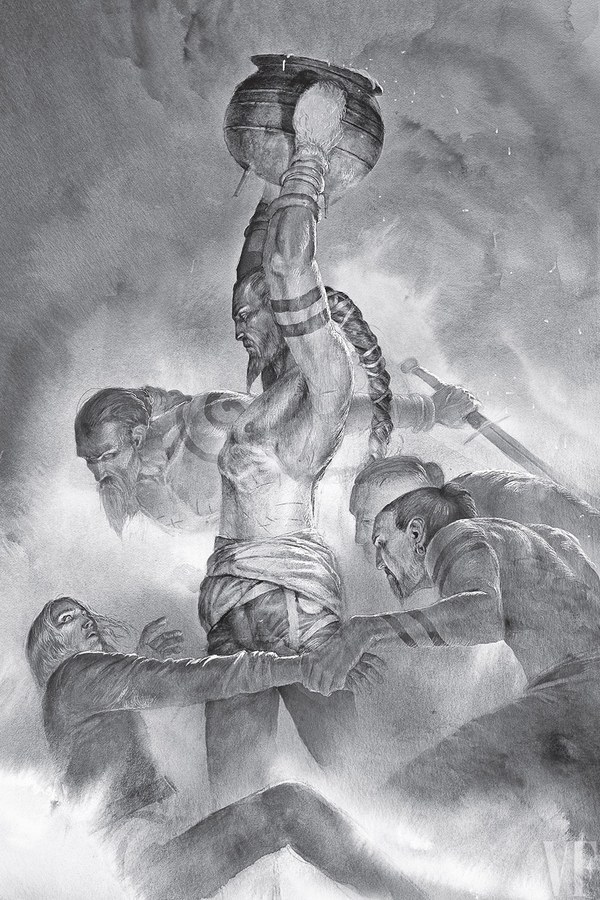This intricate black and white illustration, rendered in highly detailed pencil strokes, portrays a surreal and evocative scene teeming with mythological and fantastical elements. At the center stands a bearded man, his arms raised above his head as he holds a round pot aloft. His hands, unusually paddle-like, add a sense of otherworldly mystique. The man is clothed in a shirt with a fabric wrap around his waist and trousers, hinting at an ancient or ethereal setting.

Below him are two more figures. On the right, a man is grasping the arm of a seated woman with flowing hair, suggesting an intimate or protective gesture. She appears pensive, possibly gazing at the mysterious figure above. Clouds swirl around them, enhancing the dreamlike atmosphere of the scene.

In the midsection of the central standing man, another bearded figure appears to be flying, brandishing a sword and looking down towards the seated woman. This figure's presence within the man's torso could symbolize an inner struggle or a supernatural connection, further enriched by the surrounding clouds that obscure and reveal parts of the scene.

Additionally, behind the man who is holding the woman, another male figure emerges from the mist, adding layers of depth and complexity to the composition. This figure's indistinct form, coupled with the swirling clouds and mist, infuses the illustration with a sense of magic and mystery.

The presence of the cauldron and the mist, along with the unusual band-like appendage extending from the central figure’s head, evokes themes of magic and mythological realms. The overall scene suggests a narrative that could be drawn from a fantasy book or a metaphorical representation of cosmic or existential themes, transcending ordinary reality to capture an almost celestial tableau.